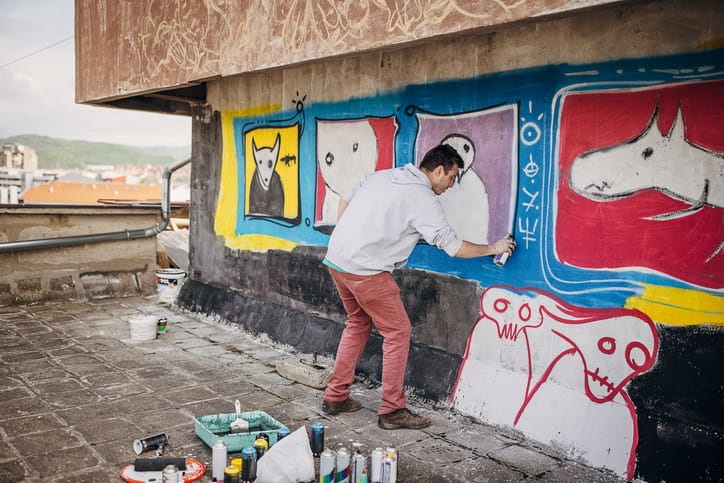In this image, a man is captured painting a mural on a large, worn concrete wall, which stretches diagonally from the middle right to the upper left of the frame. The wall is aged, with its upper portion painted beige and the lower part black, creating a stark contrast. The mural consists of four abstract panels featuring dog-like and human-skull-headed creatures in various poses and angles. The man, who is dressed in a white hoodie with a green shirt underneath, red pants, and brown shoes, is actively painting the third panel from the left. He holds a paint can in his right hand and is applying paint to the mural.

He appears to be on a surface covered with square concrete stones, likely on one of the roof levels of an abandoned building; a concrete overhang is visible above his head. To the left of the image, an array of painting supplies including cans, jars, a tray, and brushes are scattered on the ground. The background reveals rooftops of adjacent buildings, a broad rolling hill with green patches, and a glimpse of the sky to the upper left. Above the man, the remaining panels also feature intricate designs and creature imagery, all set against a blue backdrop.